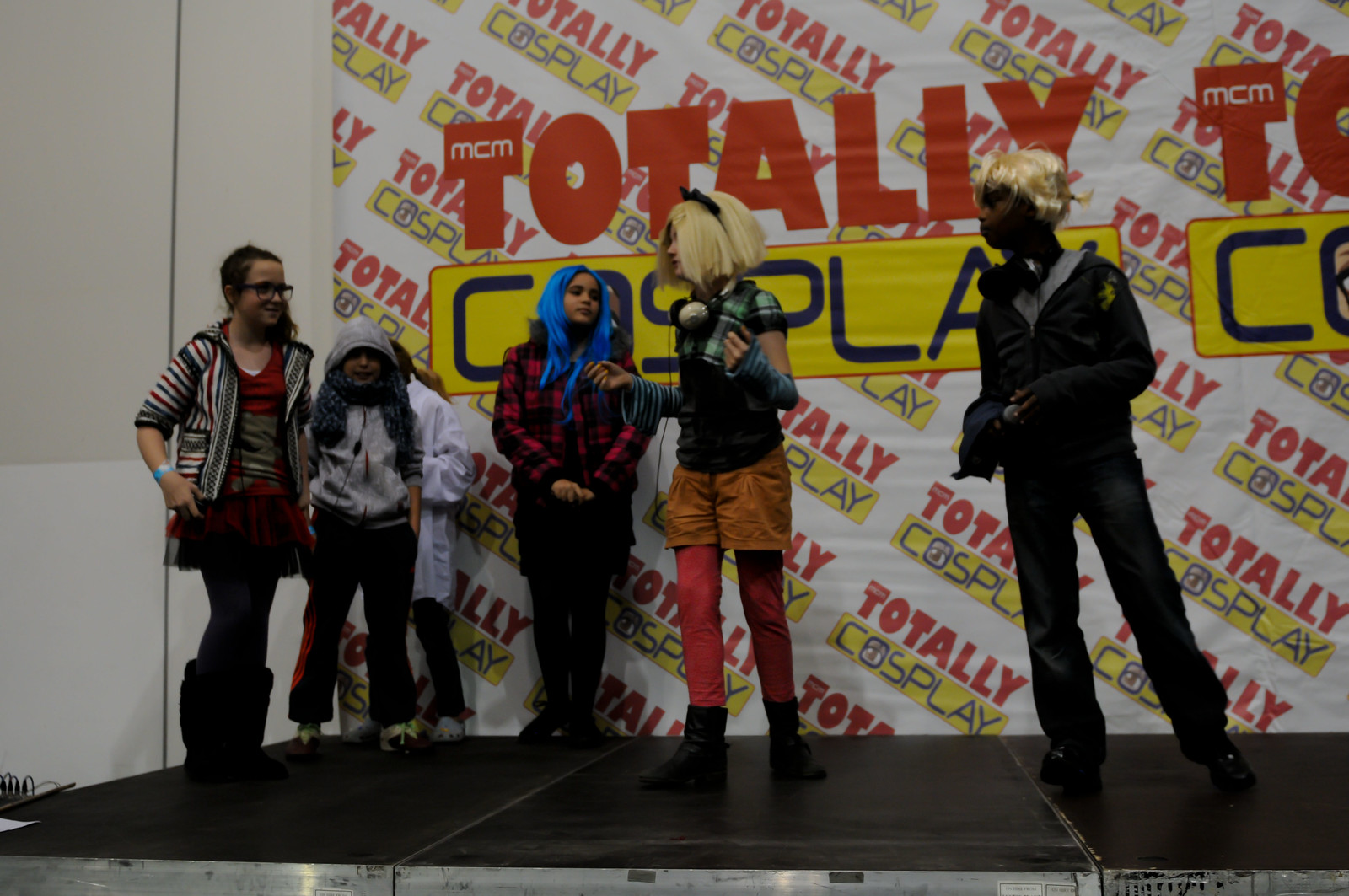The horizontally aligned image portrays a lively scene on a stage set against a large banner emblazoned with the words "TOTALLY COSPLAY" in a recurring pattern. The most prominent elements on the banner include the word "TOTALLY" in large red block letters, with "MCM" in capital white letters situated inside the "T," and a yellow rectangle outlined in red, featuring the blue-lettered word "COSPLAY." The stage itself is black and serves as the platform for six individuals, each uniquely dressed, suggestive of a cosplay event. 

On the far right stands a young African American man with short blonde hair, dressed in all black. At the center is a female with straight, short blonde hair, which appears to be a wig, adorned with a black headband. She is dressed in a plaid top with brown shorts over red leggings and black boots, and she looks to the left. 

In contrast, a group comprising three young women, seemingly just stepping onto the stage, engages with the central figures. One of these young women is wearing glasses, her brown hair pulled back, and she is attired in a striped jacket over a red T-shirt, paired with black pants and boots. Another individual, younger and with a gray hood up, has her hands in her pockets and is dressed in black pants. 

Additionally, a young girl with blue hair and another person with a hood on also populate the scene. At least one of them appears to be holding a microphone. The overall setting, with its vibrant assortment of colors—white, black, silver, red, pink, gray, blue, orange, yellow—suggests an indoor cosplay event where participants are immersed in the vivid and imaginative world of costume play.